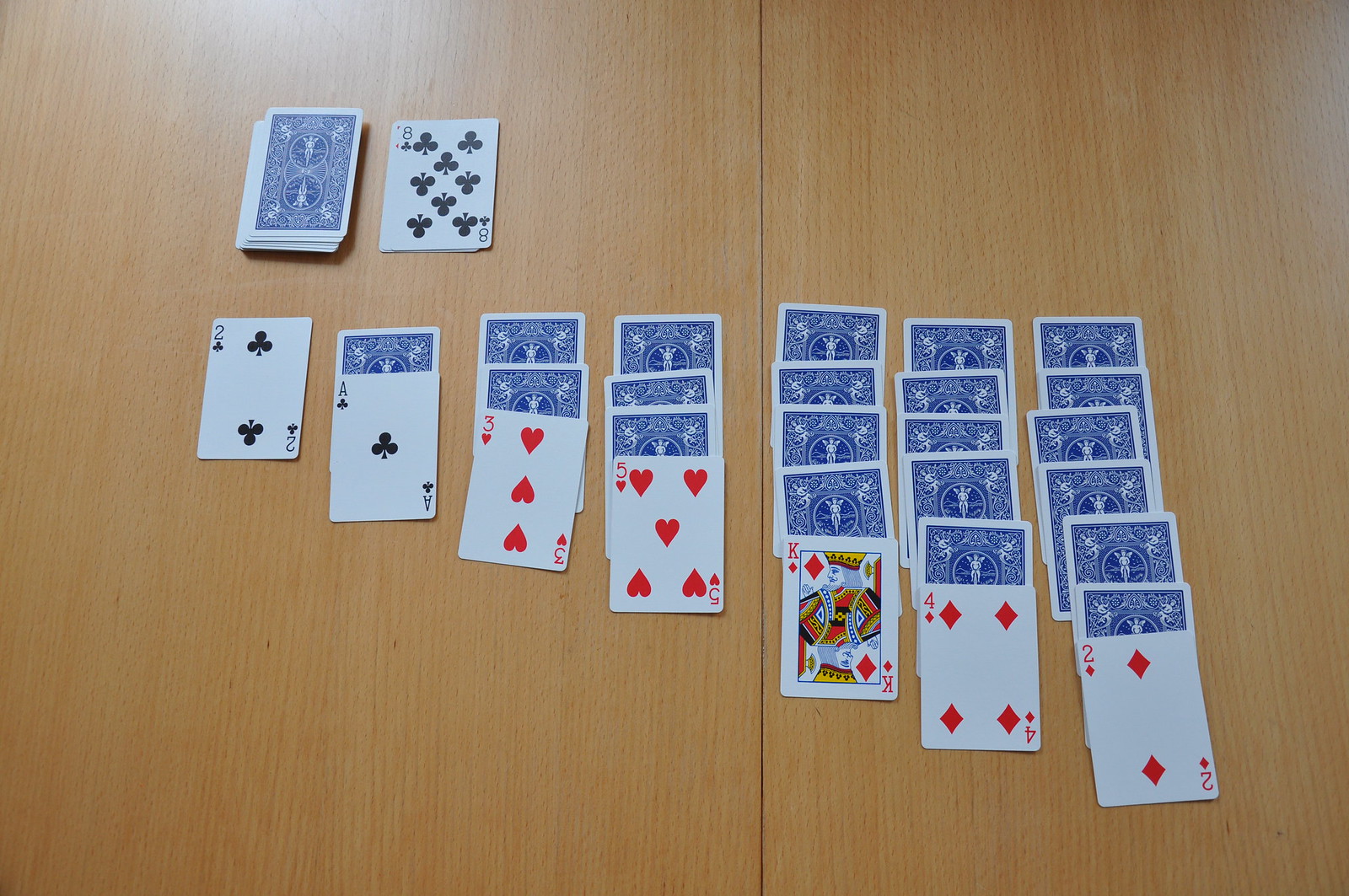In this overhead photograph, a solitaire card game is meticulously laid out on a light wood laminate tabletop adorned with a distinctive black seam running down its center. The cards, part of a standard blue deck with elegant white detailing, are arranged in cascading rows from left to right, with each subsequent row increasing by one card. The visible cards at the bottom of each column are uniquely identifiable: two of clubs, ace of clubs, three of hearts, five of hearts, king of diamonds, four of diamonds, and two of diamonds. The remainder of each row's cards are placed face down, hinting at the strategic intrigue of the game. To the left, directly above the face-up two of clubs, lies the draw pile, showing the card backs. Adjacent to this draw pile, a smaller pile of a few cards is turned to reveal the eight of clubs on top, providing a strategic edge to the player. The scene captures the essence of the classic solitaire setup, inviting the viewer into a moment of quiet concentration and anticipation.